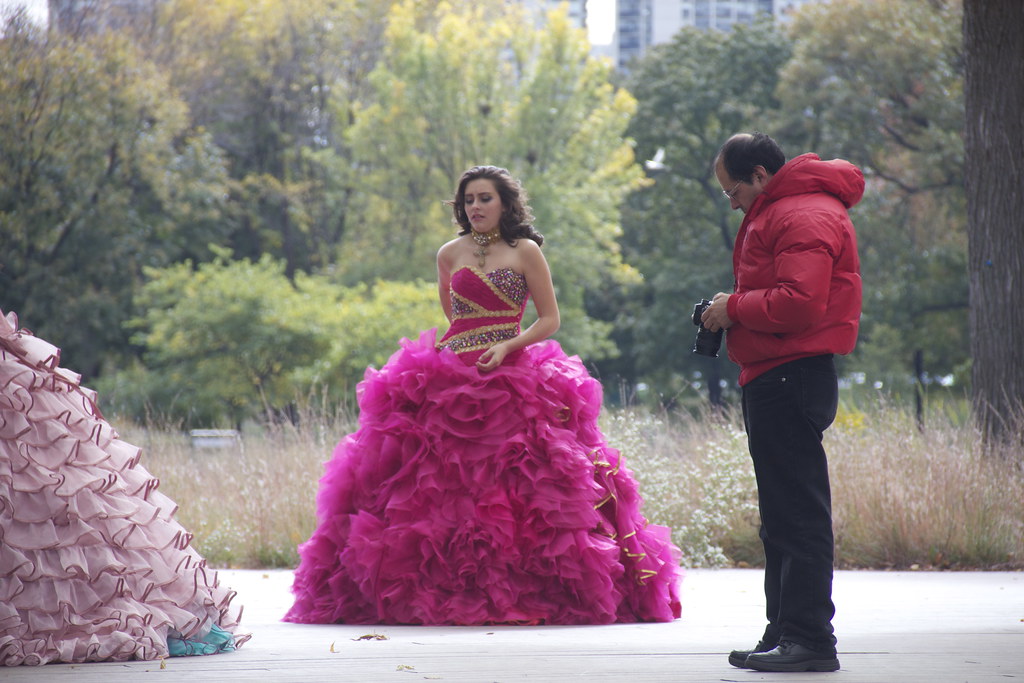In this outdoor photograph set in a public space with a paved area next to a park, the scene is populated with towering trees boasting a mix of green, yellow, and orange hues. Dominating the center-left of the image, a woman stands gracefully in an elaborate, floor-length red gown embellished with silver sequins and purple bands. The strapless and sleeveless dress cascades down into voluminous frills, giving her a princess-like appearance. Despite her fairylike attire, she seems uncomfortable, possibly due to the chilly weather hinted at by the man's thick, puffy red winter coat. He stands to the right, dressed in black pants and shoes, meticulously examining his camera. To the left of the woman, hints of another similarly extravagant dress, composed of pink and white fabric, peek into the frame. The background showcases distant tall buildings partially obscured by a line of multicolored trees and a stretch of tall grass, providing a serene and picturesque backdrop.